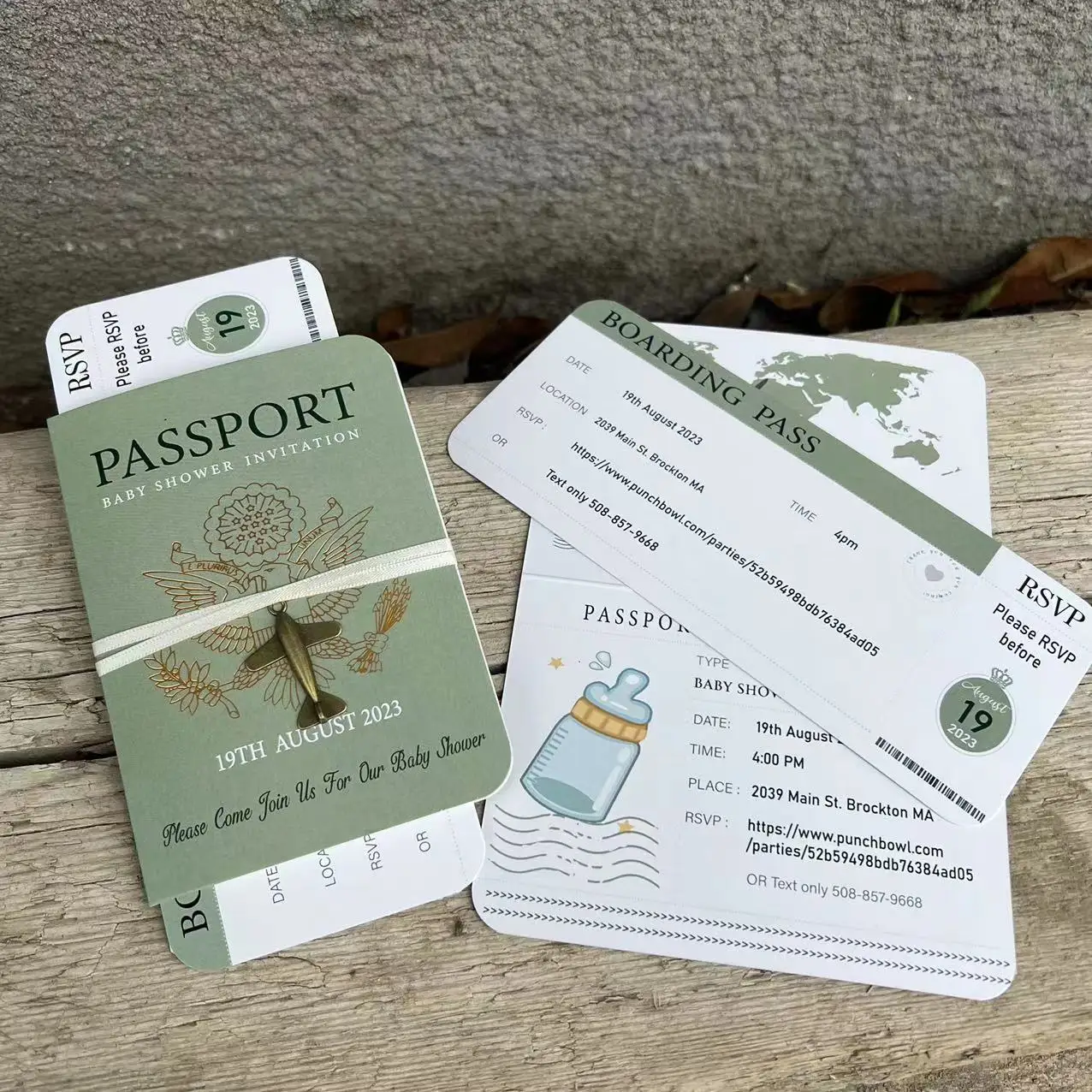The photograph depicts a baby shower invitation set styled as travel documents, laid out on a light brown wooden bench with a rough concrete wall in the background. The centerpiece is a pale olive green "passport" with black and white print. The cover features an eagle holding an olive branch and arrows, with the words "PASSPORT" and "BABY SHOWER INVITATION" in white text. A white cloth band with a gold airplane ornament secures the passport, which prominently displays the date "19th August 2023" along with the message, "Please come join us for our baby shower." To the right of the passport is a matching olive green boarding pass displaying crucial event details— the date, location at "2039 Main Street, Brockton, Massachusetts," RSVP information, and a website link for RSVP. The creative design mimics real travel documents, adding a whimsical touch to the baby shower invitation.